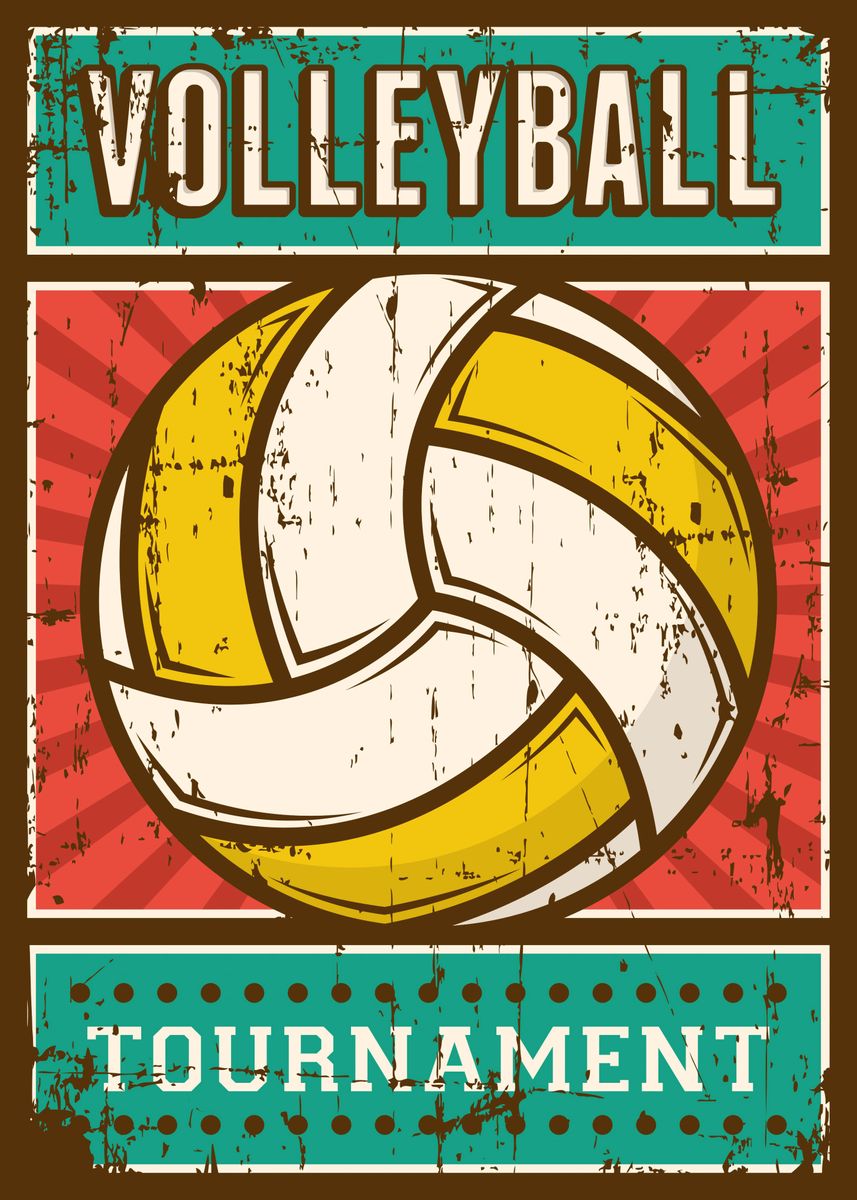This is a detailed drawing, presumably digital, of an old-fashioned metal sign for a volleyball tournament. The sign is vertically rectangular and bordered by a thin brown trim. The top features a smaller horizontal rectangle with a seafoam green (or teal blue) background and a white trim. Written in bold, capitalized white letters with black shading is the word "VOLLEYBALL."

Beneath this, there is a section filled with a red background where the focal point is a large volleyball shown in white and gold. This central element is highlighted by alternating red and dark red streams of color emanating from behind the ball, adding a sense of dynamism to the design.

Below the volleyball image is another horizontal rectangle, again with a seafoam green (or teal blue) background and white trim. It bears the word "TOURNAMENT" in the same bold, capitalized white font as "VOLLEYBALL," and the word is framed by series of brown dots both above and below it.

The sign shows signs of wear, with scratch marks and areas where the brown trim appears stretched or faded, adding to its vintage appearance.